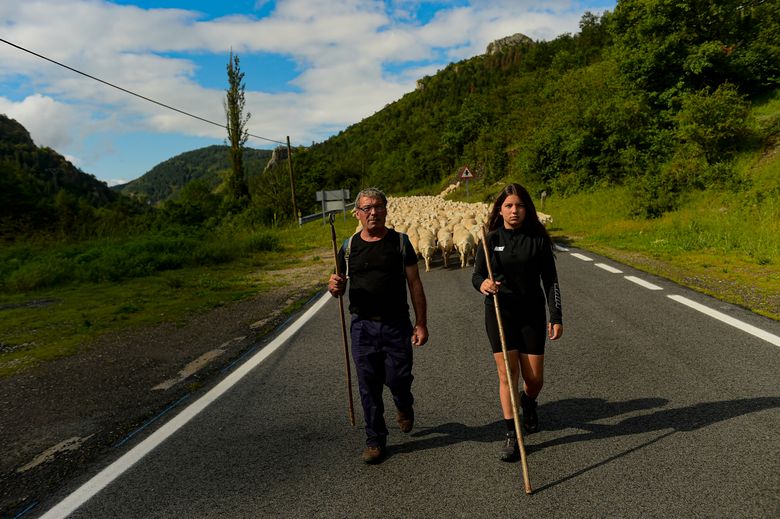In the photograph, two people, likely a father and daughter, walk down the center of a paved hillside road bordered by a continuous white line on the left and broken dotted lines on the right. The older man on the left, appearing in his 40s or 50s with gray hair and glasses, is attired in a black shirt, blue jeans, and brown shoes. He carries a backpack and holds a brown wooden staff in his right hand. Beside him, the teenage girl, approximately 13 to 15 years old, with long dark brown hair, is dressed in a black long-sleeve shirt, black biking shorts, black socks, and black sneakers, and she too holds a staff in her right hand. The pair are leading a flock of sheep, which fills the background and spans the entire width of the road, extending back into the distance. The sheep are predominantly white or off-white, all following the duo toward the camera. The landscape around them is green, with trees, grass, and a hillside extending up to the right. To the left, the road is flanked by scrub, with a valley and tree-covered hills in the background. The sky above is blue with white fluffy clouds, adding to the pastoral and serene atmosphere of the scene. Telephone poles with wires appear to stretch towards the left-hand corner of the image.